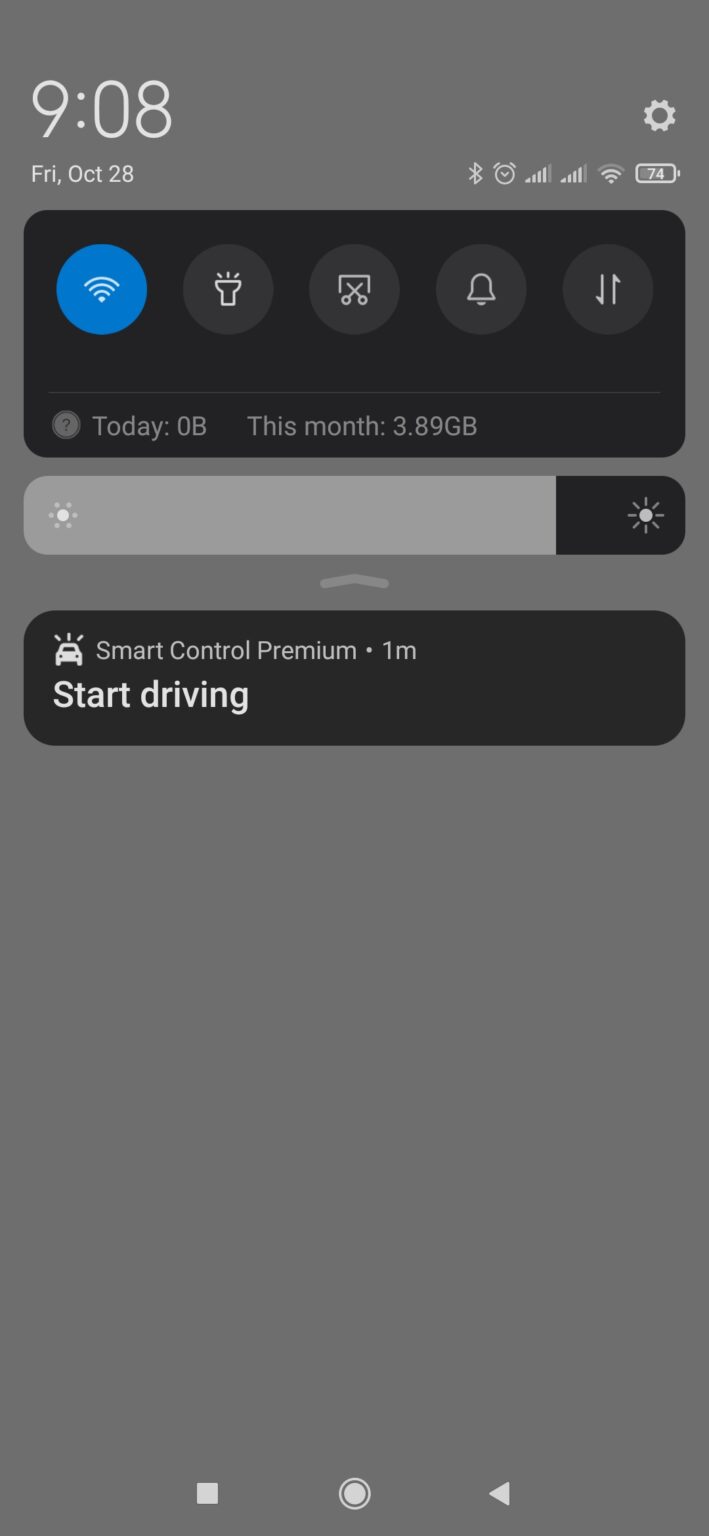A detailed screenshot captured on a smartphone shows a variety of information primarily from the notification and quick settings menu. The battery level is at 74%, and the time displayed is 9:08 AM on Friday, October 28th. The Wi-Fi is turned on, as indicated by the corresponding icon. This screenshot represents the view one would see by swiping down from the top of their phone to access the quick settings menu.

In the screenshot, several quick setting shortcuts are visible, including those for the flashlight, a scissors icon (possibly for screen capturing or another function), and an icon for reminders. However, only the Wi-Fi option is currently active. The data usage information displayed shows that no data has been used today, but 3.89 gigabytes have been consumed over the month.

The brightness slider indicates that the screen brightness is set almost to its maximum level. Below the brightness control, there is one notification stating, "Smart Control Premium, 1 minute ago: Start driving." This notification likely references a navigation app, encouraging the user to commence driving.

Overall, the screenshot provides a clear glimpse into the phone's current status, quick settings, data usage, and recent notifications.